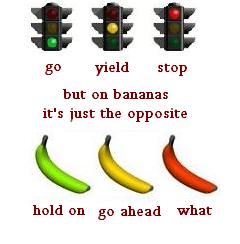This image is a comical, low-resolution digital illustration with a white background. At the top, there are three black traffic lights arranged horizontally, each with a colored light lit: green on the left, yellow in the middle, and red on the right. Underneath the green light, the text reads "go," beneath the yellow light, it says "yield," and under the red light, it says "stop." Below these traffic lights, in the same lowercase, typewriter-style font in burgundy, is the caption "but on bananas, it's just the opposite."

Beneath this caption, there are three bananas aligned horizontally with their tips pointing upwards to the right. The leftmost banana is green with the label "hold on," the middle one is yellow labeled "go ahead," and the rightmost banana is an orangey red with the label "what?" This humorous image juxtaposes the standard traffic light signals with the ripening stages of bananas, playfully noting how their color meanings are reversed. The entire layout looks neat and the text style remains consistent throughout, contributing to the whimsical nature of the illustration.